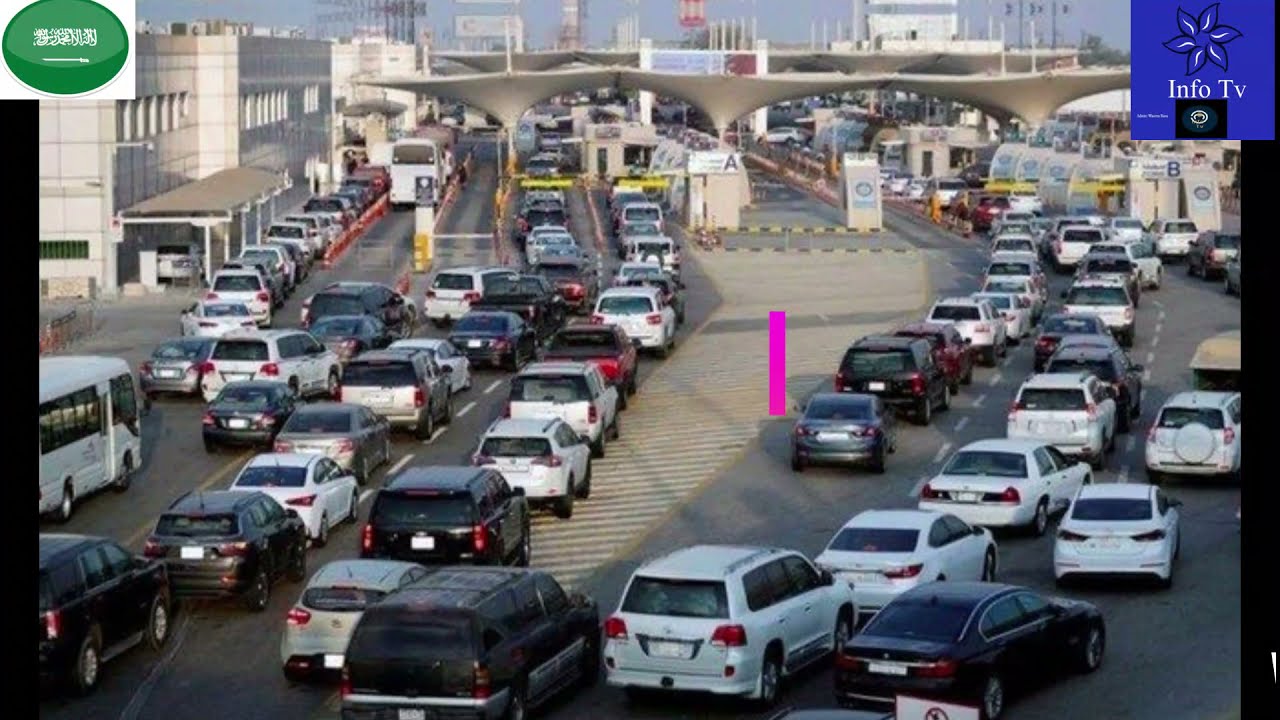The image depicts an extremely congested tollway, likely situated in an Asian city, teeming with an impressive number of vehicles, including black, white, and gray cars, SUVs, and several buses. The road is expansive, featuring at least seven to nine lanes, each thoroughly packed with waiting vehicles. Prominent in the scene are the toll booths equipped with yellow barriers that control the flow of traffic, which have uniquely designed roofs—pointed at the bottom and expanding into flat, interconnected tops. In the top left corner, there is a green circular logo with white Asian text, possibly featuring a horizontal white sword. The top right displays a blue logo labeled "Info TV" accompanied by a blue flower. A McDonald's Golden Arches logo is visible in the middle of the top section, while the background reveals several buildings under a clear sky.